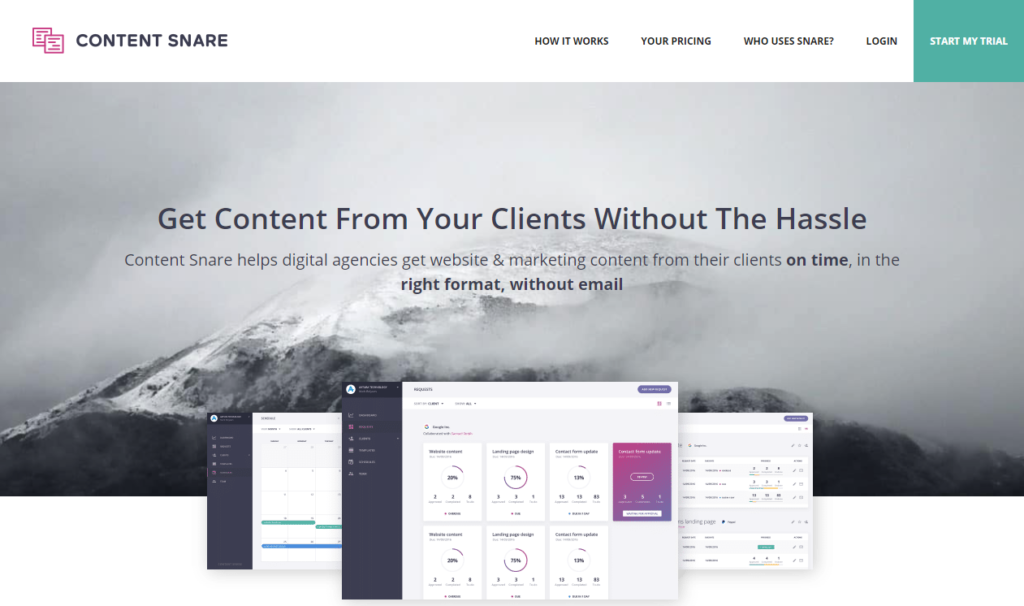The image is a screenshot displayed against a plain white background. In the upper left corner, the "Content Snare" logo is prominent, accompanied by two red flags and some white elements. To the right of the logo, several navigation options are visible, including "How it Works," "Pricing," "Who Uses Snare," as well as buttons for "Login" and "Start My Trial" in a distinctive green box.

Beneath this, a black and white photograph of a snow-capped mountain is set against a gray, smoky, and foggy sky. Overlaying this photo in bold black text is the message: "Get content from your clients without the hassle. Content Snare helps digital agencies get website and marketing content from their clients on time in the right format, without email."

Below this text is an image of a computer monitor screen. Although the specific content on the monitor is unclear, the screen features a dark navigation bar on the left side and various graphs displayed in white and purple on the right side.